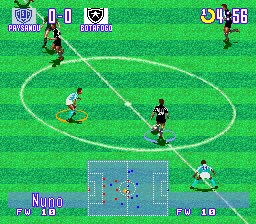This is a detailed screenshot of a soccer video game. The central focus is a close-up view of six players on the field, engaged in active play. At the bottom of the screen, there is a small rectangular mini-map displaying the entire soccer field, providing an overhead view of the players’ positions. Text on the left side of the screen reads "Nuno" alongside either "FW10" or "FW18," indicating a player’s username and character designation. The opposing side lacks a name, suggesting a match against the computer-controlled opponent, also labeled "FW10" or "FW18." The game timer shows there are 4 minutes and 56 seconds remaining, and the current score is tied at 0-0. The names of the teams are not legible, but they are the same teams that were featured in the previous match.